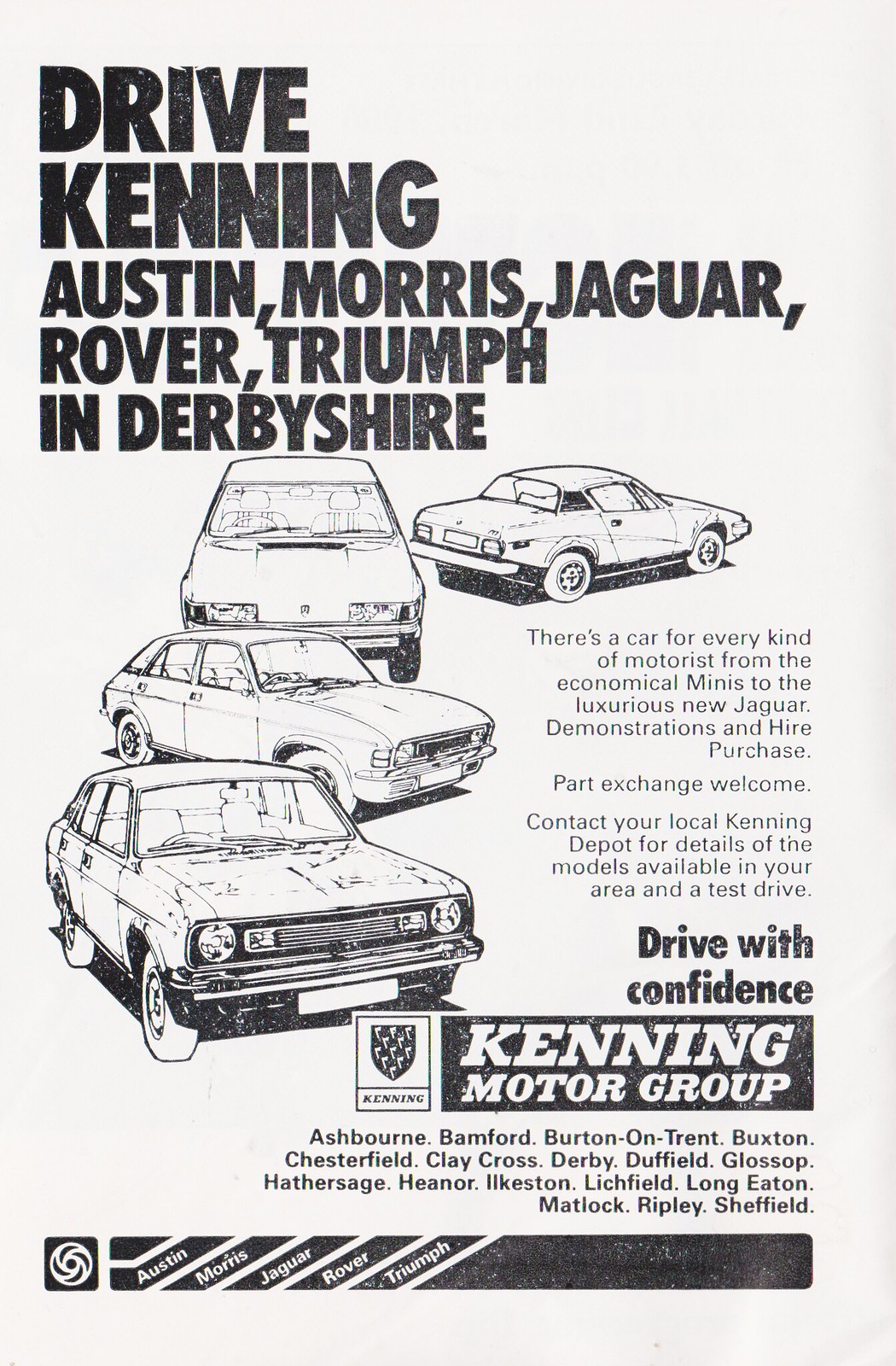The advertisement, presented in black and white and assumed to be from a British magazine, features the headline "Drive Kenning" followed by a list of car brands including Austin, Morris, Jaguar, Rover, Triumph, and Derbyshire. The top section is set against a white background with all text in black, indicating it's a promotional page for the Kenning Motor Group. The layout includes four stylized line drawings of cars: one prominent car in the center and three others arranged vertically on the left side. These illustrations depict various car types such as a Triumph sports car, a family car, a compact car, and a sedan, emphasizing the range of vehicles on offer.

The advertisement copy highlights that there is "a car for every kind of motorist, from the economical Minis to the luxurious new Jaguar." The ad also mentions services like demonstrations and hire purchase options, along with part exchange offers. Prospective buyers are encouraged to "contact your local Kenning Depot" for model availability and test drives. The motto "Drive with Confidence" appears prominently near the bottom, accompanied by the Kenning Motor Group's coat of arms and shield logo.

Below the logo, a comprehensive list of cities where Kenning Motor Group operates is provided, including Ashbourne, Bamford, Burton, Buxton, Chesterfield, Clay Cross, Derby, Duffield, Glossop, Heage, Heanor, Ilkeston, Lichfield, Long Eaton, Matlock, Ripley, and Sheffield. Along the bottom of the page, a black strip features the names of prestigious car brands like Jaguar, Rover, and Triumph, underscoring the group's extensive offerings.